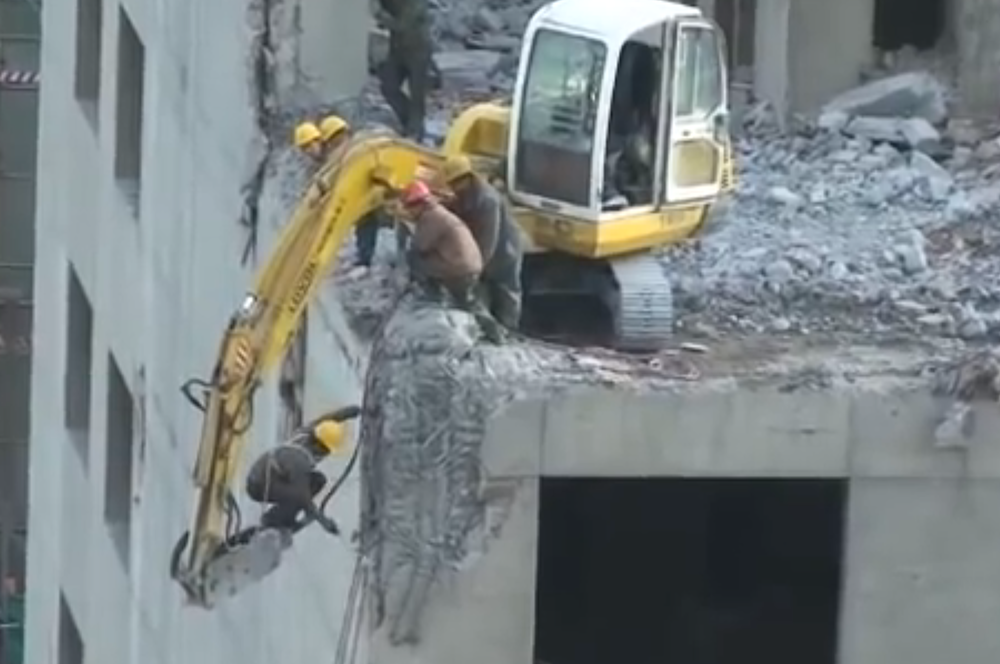This image, grainy and intensely detailed, captures a perilous scene at a high-rise construction or deconstruction site from an elevated perspective. The focal point is a partially deconstructed or under-construction building with concrete debris scattered across its rooftop. A large bulldozer, possibly a crane, is positioned precariously on the roof, its arm extending downward off the edge. One worker, clad in a yellow hard hat, sits dangerously close to the edge of the machine, working on rebar at the building's precipice. Above him, another worker with a red hard hat peers down, overseeing the activity below. Around them, up to five workers, all wearing hard hats, safety vests, and harnesses, navigate the rubble-strewn surface. The building's windows are hollow and unfinished, contributing to the sense of instability and incompleteness. The open driver compartment of the heavy machinery and the unsecured nature of the rooftop atmosphere exude a sense of danger and urgency, underscoring the chaotic environment of the site.